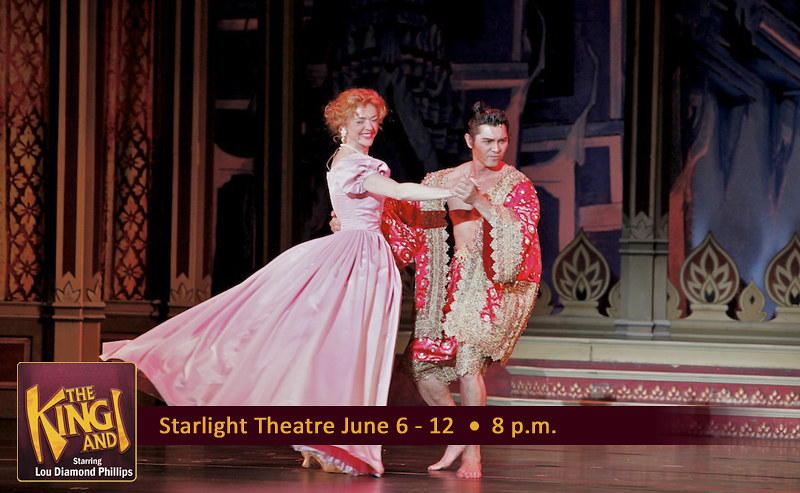The image is a detailed photograph capturing an on-stage performance of the musical "The King and I." In the lower left-hand corner of the image, there is a red square bordered in gold with bold print that reads "The King and I," followed by "Starring Lou Diamond Phillips" in white print. Extending from the middle right side of the square, a maroon banner with gold letters states, "Starlight Theater, June 6th-12th," with an adjoining circle indicating an 8 p.m. showtime.

Central to the photograph, a young woman of Caucasian descent and a man, likely of Filipino descent but portraying an Indian character, are captured mid-dance. The woman wears a floor-length, poofy-sleeved pink dress with glimpses of white fabric and gold or yellow heels visible beneath its hem. Her hair is short, curled, and blonde or reddish blonde, styled up, and she beams with a closed-eye smile as she extends her right arm forward. The man's right arm is around her waist, his left hand holding hers, and he is barefoot with dark black hair pulled into a bun atop his head. He wears a lavish red and gold robe paired with shorts, his chest exposed.

The stage backdrop features walls on the left side, giving an indoor impression, while the right side displays a palace-like structure, as if the characters are on a balcony. This evocative scenery enhances the visual narrative of the performance, transporting the audience into the world of "The King and I."